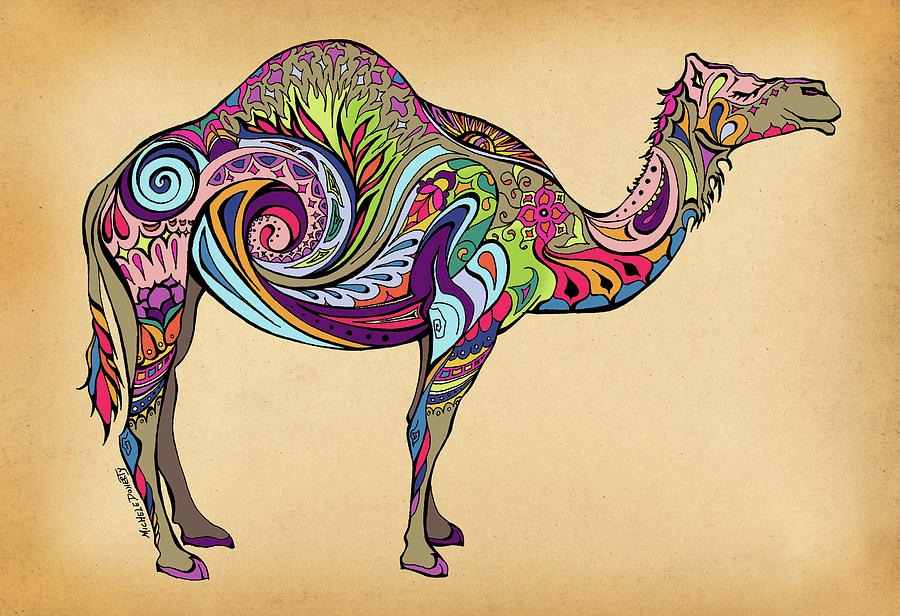This is an artistic illustration of a one-humped camel, facing left with a serene smile and closed eyes, set against a simple tan background. The camel's body is adorned with vibrant, psychedelic patterns and swirls in striking colors such as blue, purple, red, pink, green, and yellow. Notable details include its pink-painted ear and eye, and an orange butterfly near its face. The camel's tail displays a gradient of orange, red, and blue hues, matching the colorful swirls that cascade down the length of its body, almost enveloping its back left and front left legs. The hooves are painted pink, adding to its whimsical appearance. The artwork is signed near the back leg by the artist, Michele Doherty. The overall impression is one of a lively, groovy, and visually stunning piece, blending vintage charm with modern vibrancy.